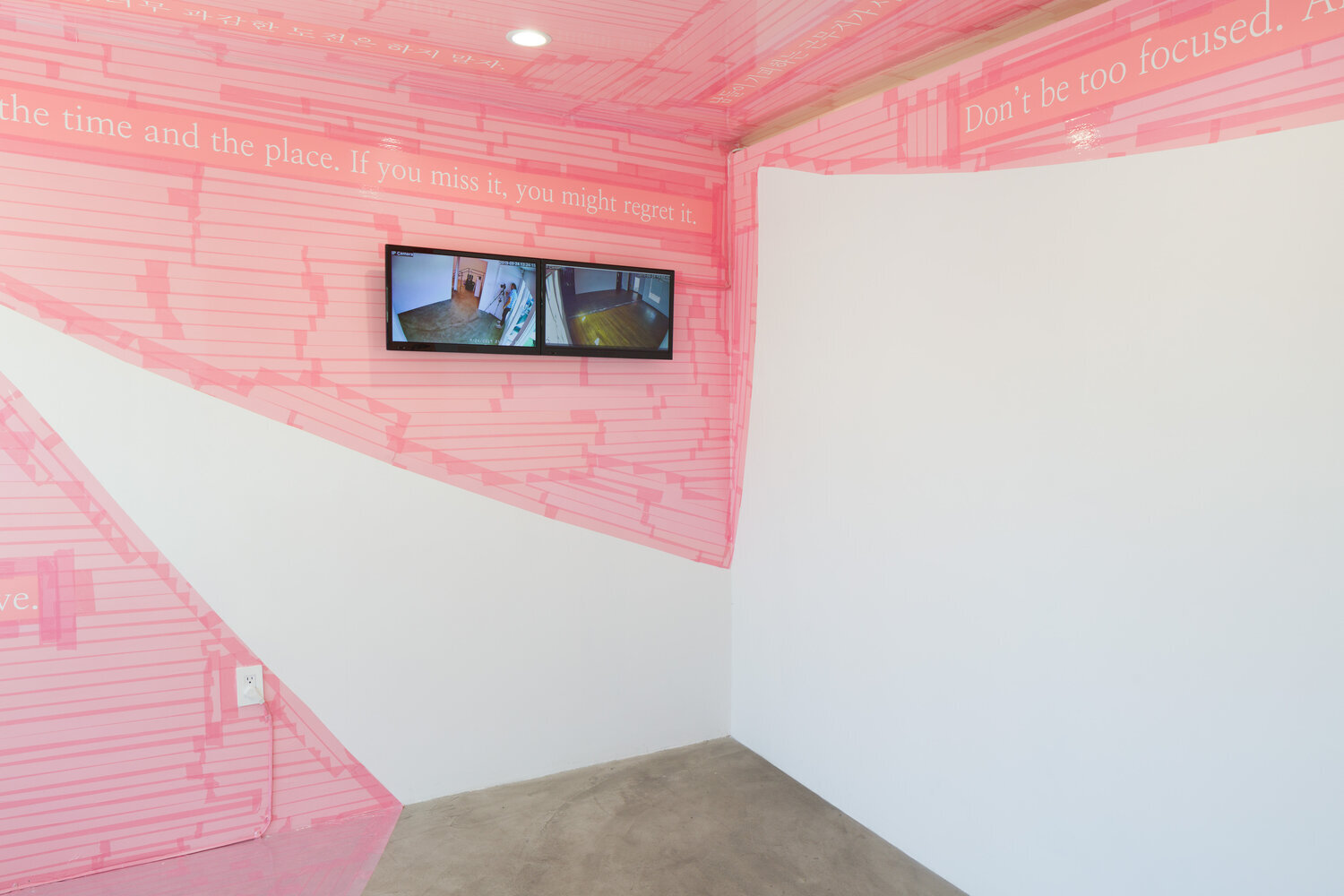This color photograph, oriented horizontally, captures an empty room with a white and pink interior. The room's corner is positioned centrally in the image, flanked by two walls that meet the ceiling above. The white walls are accented with a diagonal pattern of pink lines, creating a striking visual effect on the lower left side, upper left side, ceiling, and upper right side of the room. The pink sections feature defined brush strokes, lending a tactile quality to the scene. Two white text blocks are visible; the wall on the left displays the phrase, "the time and the place. If you miss it, you might regret it," while the upper right corner reads "don't be too focused," with additional text partially obscured. Below the text on the left wall, two monitors, reminiscent of a security setup, are positioned side by side, showcasing various images. The floor beneath them is covered with a marbled brown tile, adding texture and warmth to the minimalist design. This photograph blends elements of photographic realism with a touch of abstract art, hinting at an art installation or an unfinished room awaiting further decoration.